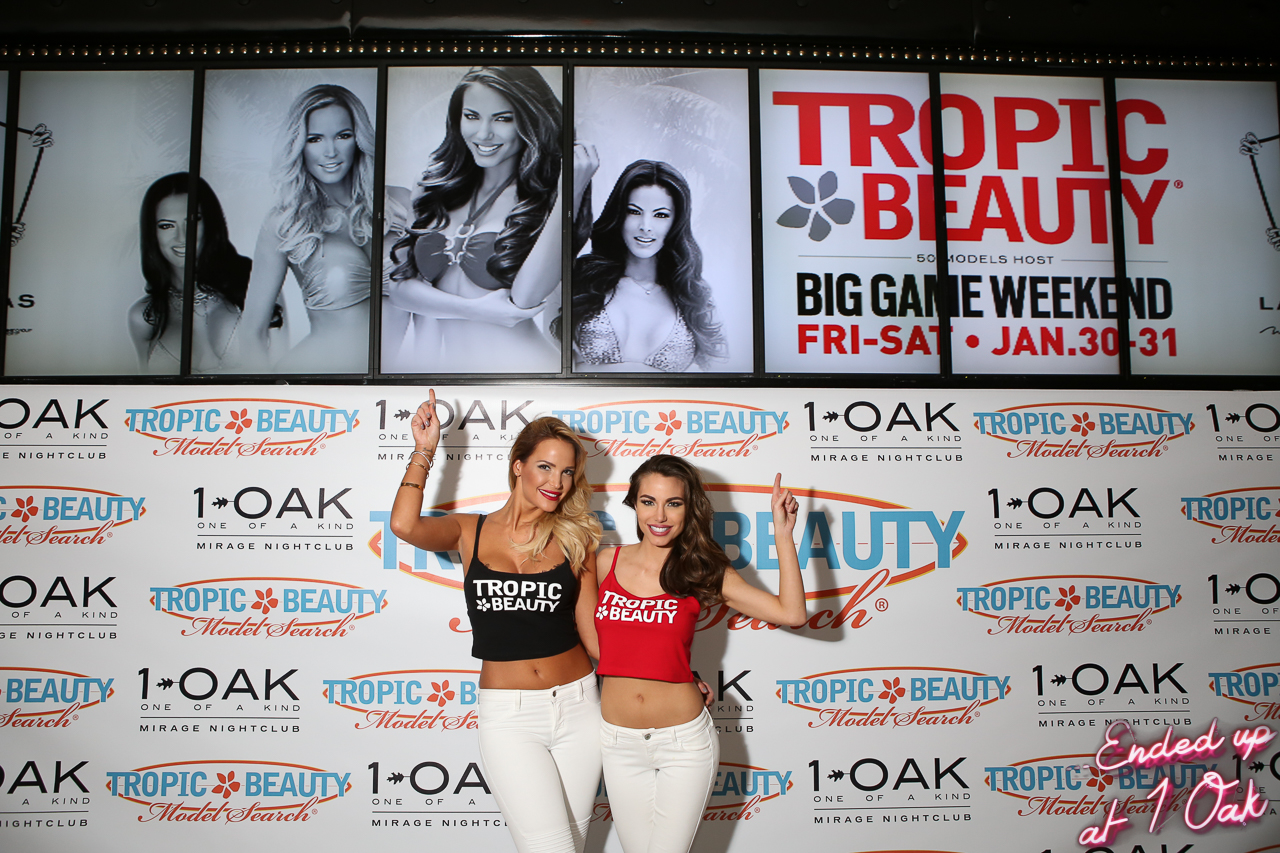In this vibrant and dynamic photograph, two women are seen standing in front of a large advertisement wall while pointing up at a striking poster above them. The wall behind them is awash with branding for Tropic Beauty in bold orange and blue colors, further accentuated by a separate ad for One Oak, One of a Kind, Mirage Nightclub. Central to the image is a black-and-white poster of four women, two of whom appear to be the very same women posing below. The advertisement prominently announces "Tropic Beauty" in red letters, followed by "Big Game Weekend" on Friday and Saturday, January 30-31. Both women are dressed in eye-catching cropped tank tops with "Tropic Beauty" emblazoned in white lettering—one top is red and the other is black. Their fashionable attire is completed with tight white jeans that highlight their stylish look. One woman has long brown hair cascading over her shoulder, while the other sports long blonde hair in a similar fashion. In the photograph's bottom right corner, a note reads, "Ended up at One Oak," tying the entire scene to the vibrant nightlife they are promoting.